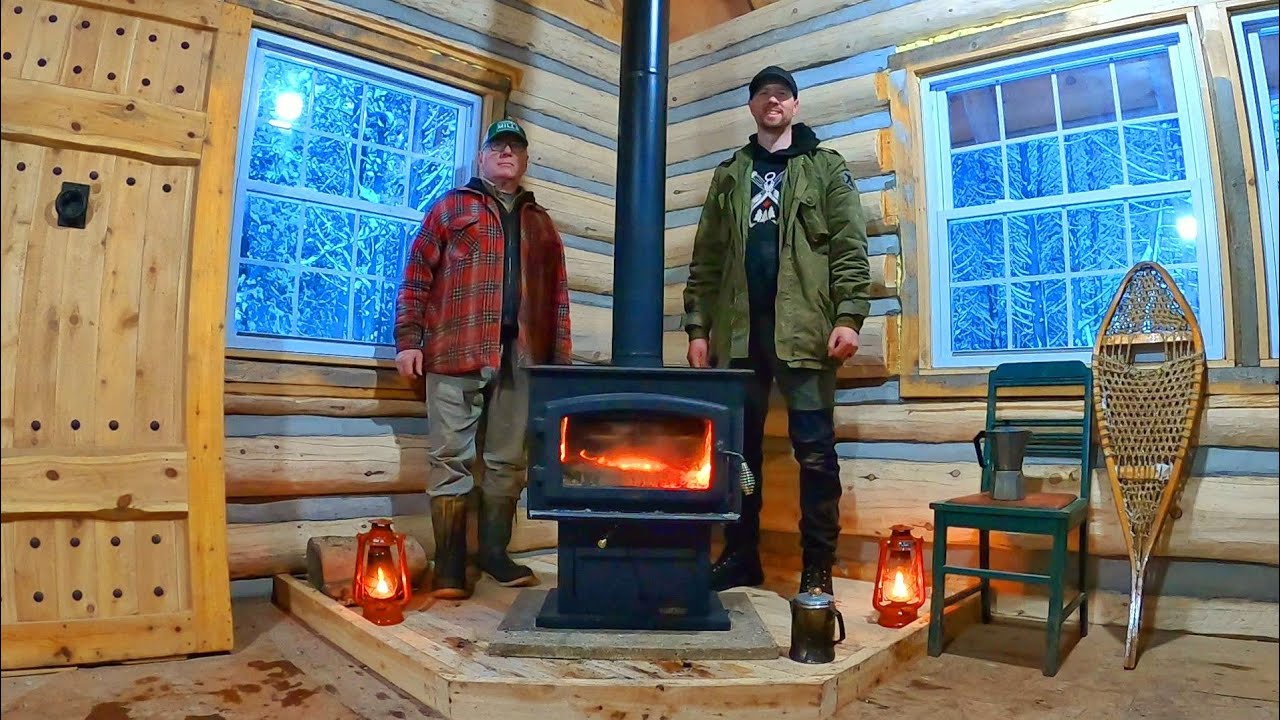In a cozy, well-lit log cabin with light-colored wood walls, two men stand on either side of a brightly illuminated old wood-burning stove, which sits on a raised platform. The younger man on the right, wearing a green jacket, black hat, black t-shirt, black pants, and black boots, smiles warmly at the camera. The older man on the left sports a red flannel jacket, a green hat, khakis, glasses, and boots. Each man is flanked by a red lantern emitting a warm glow. Among the rustic details, an old teapot rests on the corner of the stove, and a green chair with another teapot or coffee pot perched on its seat sits to the younger man's right. Leaning against the right window is an old-style woven snowshoe, while a pair of snow boots rests against the left window. Through both windows, one can glimpse the frozen branches of trees outside, encapsulating the wintry setting. A wooden door with a hook in the center adds to the quaint charm of the cabin interior.